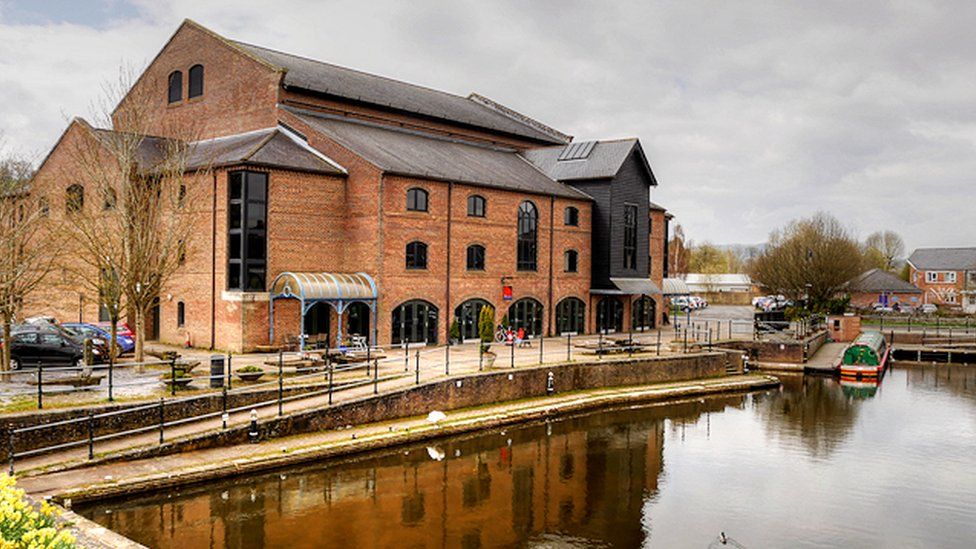The image portrays a large, orange brick building occupying almost an entire block. The structure prominently features black-framed, arched windows and spans three stories in the front. Towards the back, it rises even higher, suggesting a total of three to five floors. An inclined roof with additional windows indicates more space above the third floor. The building's facade includes four small archways, possibly entrances or windows, on the ground level. Adjacent to the main structure, a section with a different color and its own roof, possibly an addition, extends to the right. 

In the foreground, a calm, brownish body of water, likely a lagoon or lake, is present, with a dock area leading to it. Parked nearby is a tour boat. A walkway extends from the water to the building, flanked by some trees, including a few bare ones. To the left of the building, cars are parked against a backdrop of more barrack trees. The right side of the image features additional structures and trees in the distance, and another little dock with a boat moored. The overcast, gray sky casts a gloomy ambiance over the scene.